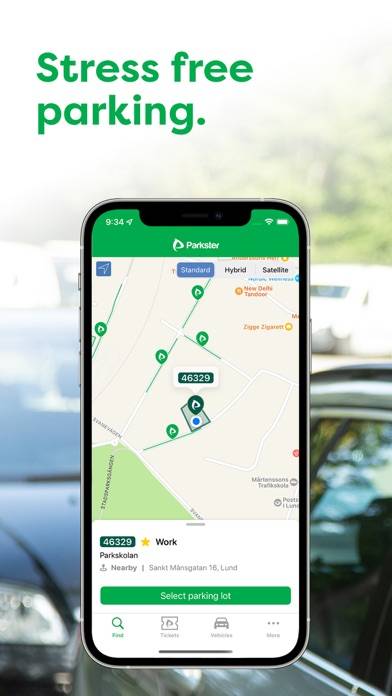This portrait-format image promotes the Parkster app, a mobile application designed to facilitate stress-free parking. 

At the top of the image, the slogan "Stress-free parking" is prominently displayed in bold green lettering on the left. Below this tagline, a detailed depiction of the app in action is shown on a black mobile phone.

The phone's screen starts with a green banner at the top, displaying essential information: 
- On the left, the time reads 9:34 in white numbers alongside a white icon.
- In the center of the green banner, the word "Parkster" appears next to the Parkster icon (a 'P' logo).
- On the right, the banner shows a connectivity strength symbol and a full battery icon.

The main display of the phone screen is dominated by a map, reminiscent of Google Maps, marked with six "P" icons indicating parking locations. Of these, five are in light green and one is in dark green. This suggests various parking spots scattered throughout the area, most likely within the city of Lund, Sweden.

Beneath the map, a white section of the screen provides further details: 
- A green banner displays the number 46329, alongside a gold star and the word "work."
- The text "Parkskolan" is listed beneath, indicating a specific location.
- Further down, "Nearby Sankt Mangarten 16 Lund" confirms the geographic focus on Lund, Sweden.

At the bottom of the app interface, another green banner reads "Select parking lot" in white text. Below this, four interactive icons are present: a magnifying glass for search, a ticket icon, a car icon, and three dots labeled "more." The text under these icons, written in Swedish, presumably provides additional functionalities related to the app.

The background of the advertisement is a blurred scene of cars lined up in a traffic jam, featuring a black car and a silver car, emphasizing the convenience and relief the Parkster app offers in such congested situations.